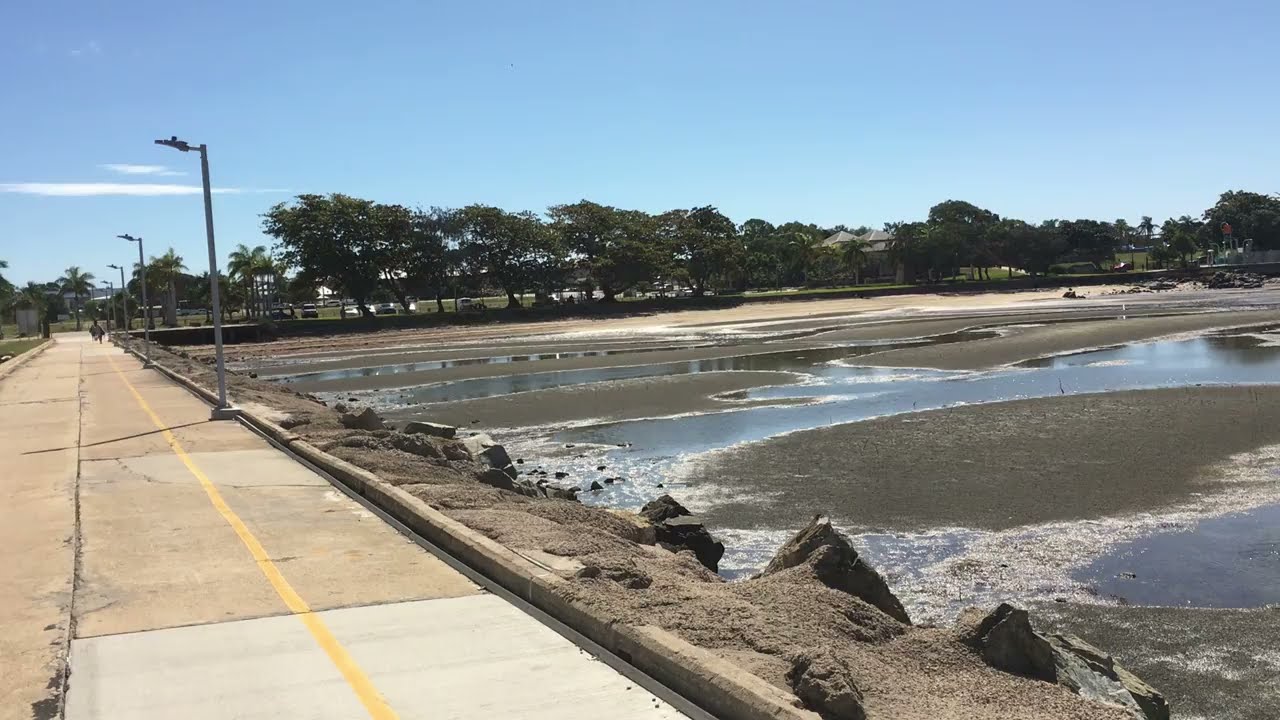This image captures an outdoor scene featuring a park area with a pathway that extends to the left. The pathway, possibly a combined pedestrian and bike path separated by a yellow line, is lined with lampposts. Adjacent to the path on the left is a wide walking area with light poles extending down its length. On the right side of the path lies a rocky, bouldery area that dips into what appears to be a shallow or dried-up body of water with numerous mounds of dry ground protruding from it. This area resembles a sandbar or wetland at extremely low tide, with gray sand interspersed with small pools of water, reflecting the pale blue sky above. Towards the far right, there is a very small, man-made-looking beach with some rocks and a couple of people sitting, likely due to the low water levels. In the background, a row of trees, some buildings, palm trees, and a few gazebo areas can be seen, along with a parking lot with cars. The sky, mostly clear with long, flattened clouds on the left side, adds to the serene atmosphere of the scene.